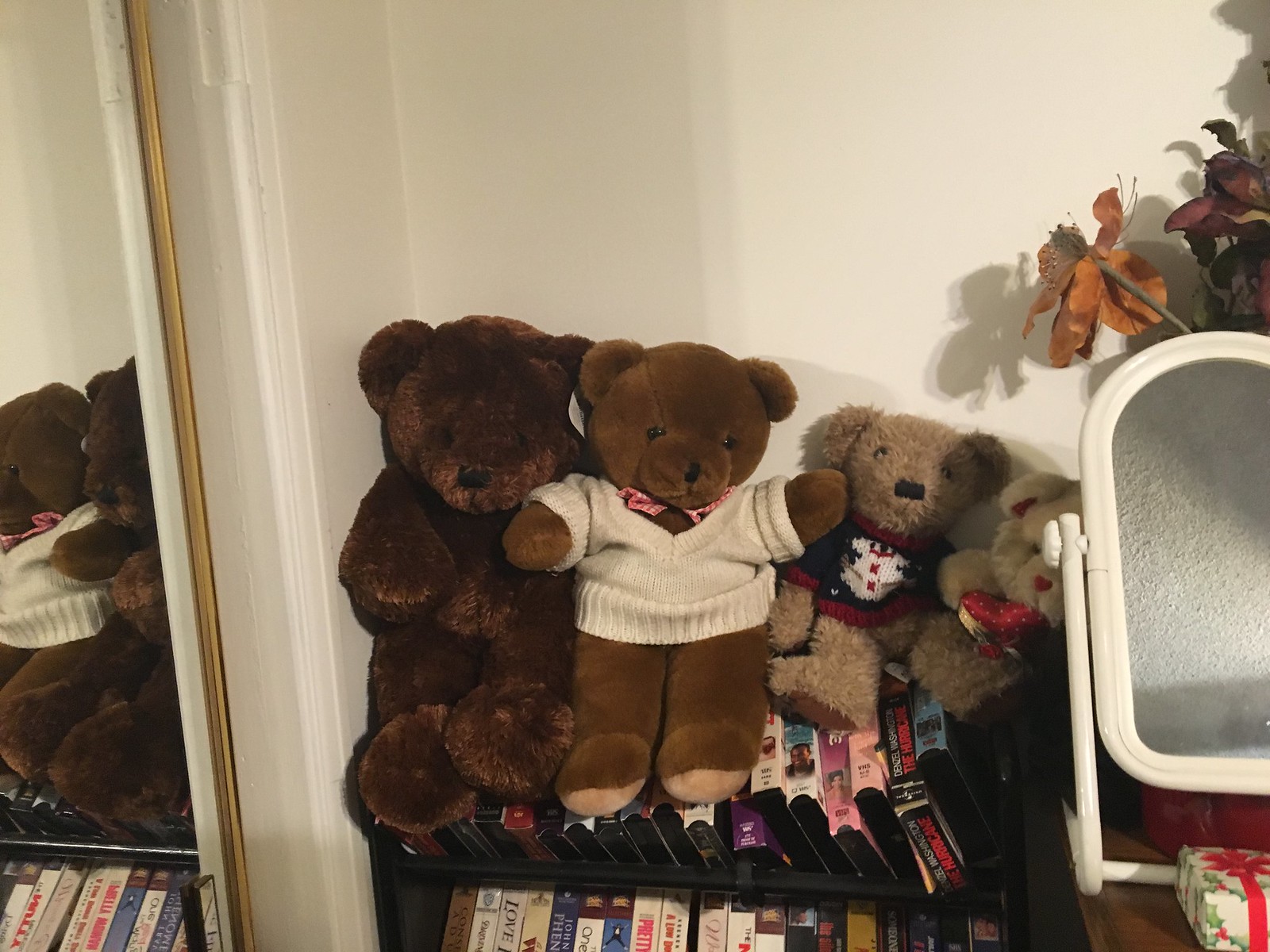The photograph captures a cozy, nostalgic interior corner, primarily showcasing a collection of four teddy bears organized by size from left to right on a black shelf designed for VHS tapes. The largest teddy bear, dark brown, sits on the left, followed by a slightly smaller teddy bear in a white sweater. Next in line is a medium-sized teddy bear with a blue, red, and white sweater featuring a snowman design and lighter brown fur. Completing the row is a small teddy bear, lighter in color, holding a red heart. All the bears have distinctive black noses and eyes. This charming row of teddy bears sits atop a fully stocked row of VHS tapes, evoking a sense of nostalgia. To the left of the shelf, a glass closet door with a mirror reflects the adorable scene of the teddy bears. On the right, a stand mirror with a white frame angles towards the ceiling, accompanied by a florally decorated side table and a vase of dried flowers, adding a vintage touch to the setting. All these elements are set against a plain white wall, with shadows cast by the objects, highlighting the room’s quaint and sentimental atmosphere.